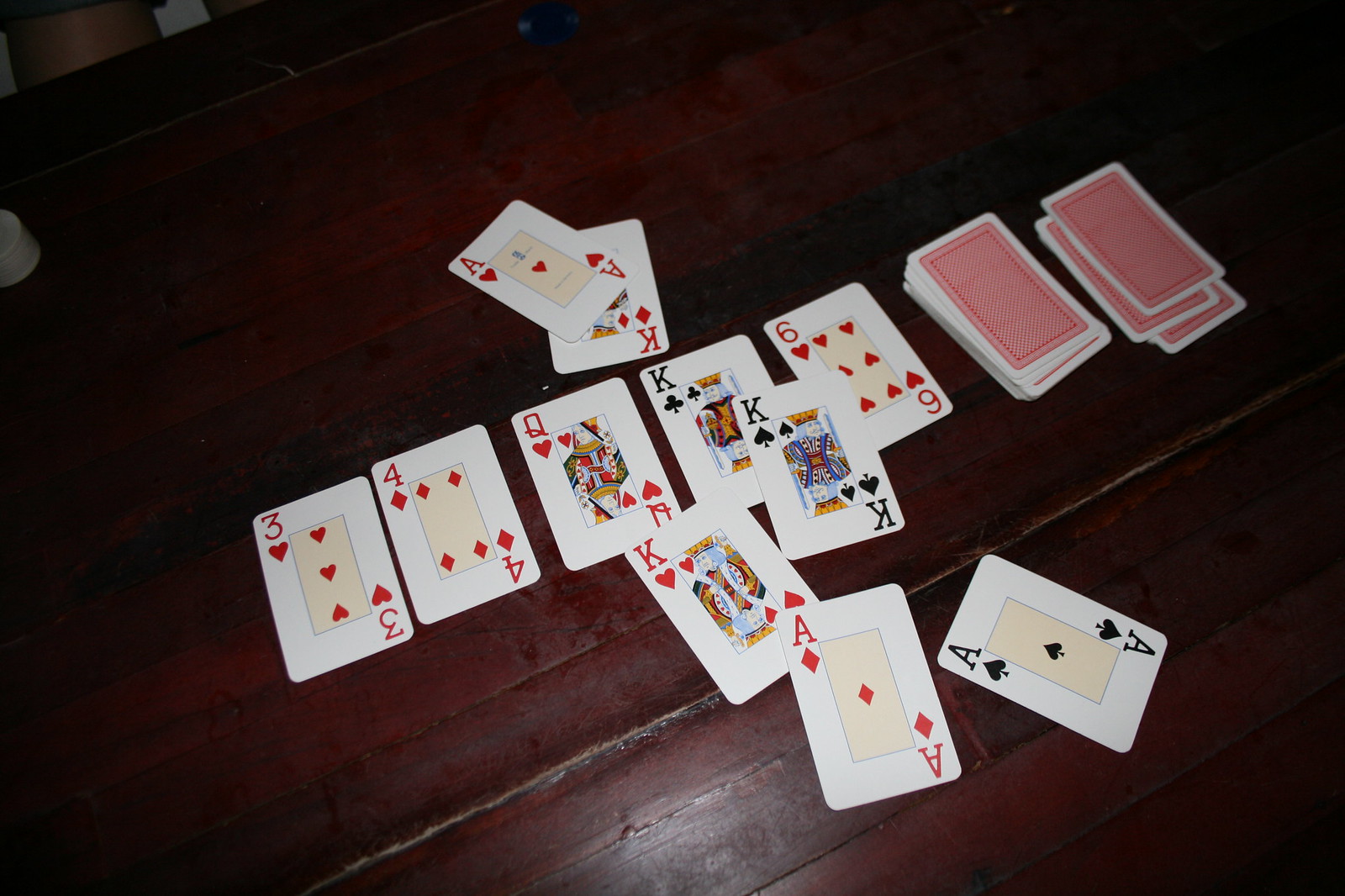The image captures an old, well-loved table, its surface polished to a glistening shine from years of waxing. The table is sparsely populated, featuring only a poker chip in the background and a spread of playing cards arranged strategically in the foreground. 

At the center of the table are three sets of faced-down cards, suggesting the initiation of a card game. In the middle row, a line of uncovered cards reveals a sequence: the three of hearts, four of diamonds, queen of hearts with a king of hearts attached, king of clubs with a king of spades trailing, and six of hearts. The pattern continues with an ace of diamonds following the king of hearts, indicating careful card placement as part of the gameplay.

Prominently displayed on the closest side of the table is an ace of spades, while the opposite side hosts an ace of hearts paired with a king of diamonds. The intricate and somewhat mysterious arrangement hints at a complex card game in progress, involving strategic combinations and potential flushes, inviting curiosity about the unrecognized game being played.